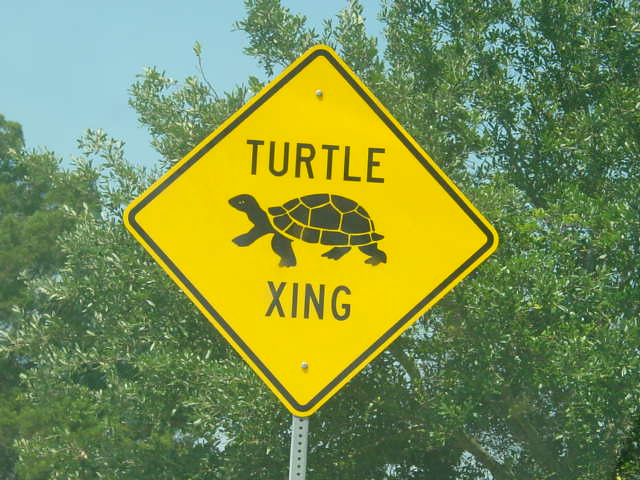This is a low-resolution photograph of a traditional American street sign, positioned in a diamond shape. The sign is yellow with a black border and features a black illustration of a turtle with its right front foot raised, as if walking leftward. It reads "TURTLE X-ING" in all capital letters. The sign is mounted on a silver perforated signpost with visible screws or bolts at the top and bottom. The background consists of dense, leafy green trees with clear blue sky peeking through, occupying most of the upper part of the image. No clouds or other objects are present, creating a simple and straightforward composition focused primarily on the sign and the natural backdrop.